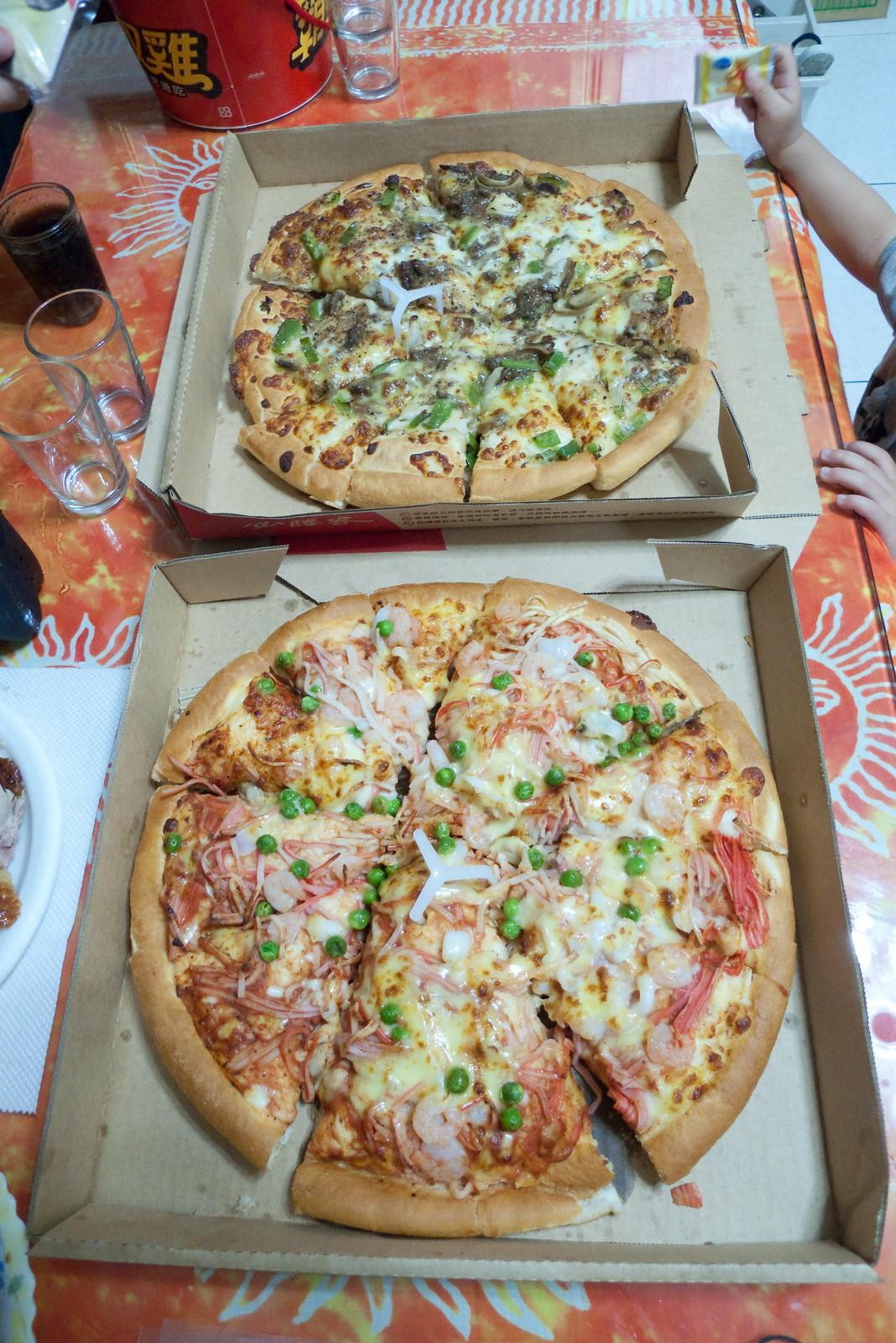The image depicts two pizzas in their respective brown pizza boxes, positioned on a vibrant, sunflower-patterned tablecloth in shades of orange and white. The upper pizza features a thick, brown crust adorned with green peppers, mushrooms, onions, a generous layer of cheese, and possibly spinach, embodying a veggie lover's delight. The lower pizza showcases a similarly thick crust, topped with yellow cheese, onions, green peas, and shrimp, accompanied by a rich red sauce that peeks through the toppings, suggesting a more eclectic combination of flavors. To the left of the pizzas, there are empty drinking glasses and one glass containing a dark beverage. Slightly rightward, the eager hands of a child can be seen, seemingly reaching toward the tempting pizzas, adding a touch of anticipation to the scene.